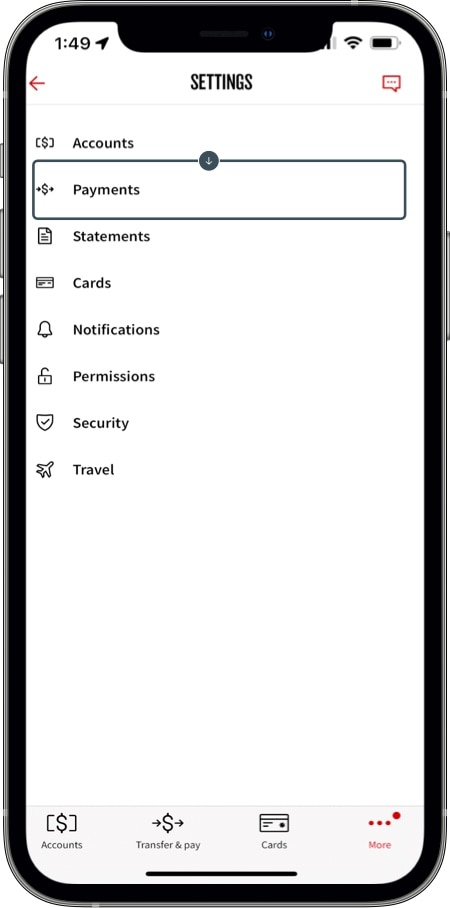The image displays a detailed user interface of a mobile application.

**Header Section:**

- **Top Left:** The number "149" is displayed.
- **Navigation Symbol:** A black, slightly diagonal arrow pointing towards the upper right indicates the user's current location.
- **Top Center:** The word "SETTINGS" appears in all capital letters using a bold, block-like font (similar to Impact).
- **Top Right:** 
  - A maroonish pink message bubble with three dots inside, indicating notifications or messages.
  - A left-hand arrow of the same maroonish pink color is also present.
- **Divider:** A thin line separates the header from the main content.

**Main Content:**

- The main section is a menu with the following options listed:
  1. Accounts
  2. Payments (currently selected, indicated by a dark gray border around it)
  3. Statements
  4. Cards
  5. Notifications
  6. Permissions
  7. Security
  8. Travel
- **Top Center of the Main Section:** A small filled dark gray circle with a white downward-pointing arrow.

**Bottom Navigation Bar:**

- **Left Icon:** A black dollar sign, labeled "Accounts."
- **Middle Icons:**
  - A money symbol with a left-pointing arrow and a right-pointing arrow labeled "Transfer and Pay."
  - An icon of a credit card labeled "Cards."
- **Right Icon:** 
  - Three small pink dots arranged vertically.
  - A larger pink dot to the upper right.
  - The word "More" in pink font underneath.

This detailed description captures the visual and functional elements of the user interface depicted in the image.